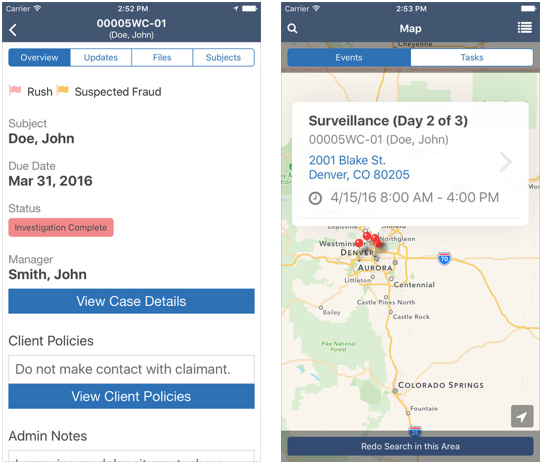The image features two smartphone screenshots displayed side-by-side. 

The left screenshot appears to be a page from a case management or investigative application. The phone's status bar at the top displays the time as 2:52 PM and shows a fully charged battery icon. Below the time, the screen lists the case ID as "00005WC-01" with the name "Doe John" in parentheses directly underneath. This section is followed by four tabs labeled "Overview," "Updates," "Files," and "Subjects." Towards the top left corner, beneath this header, there are two flagged items: "Brush" marked with a pink flag, and "Suspected Fraud" marked with a yellow flag. Further down, it details the subject as "Doe John," with a due date of March 31st, 2016. The status of the case is indicated as "Investigation Complete" in bold red text and highlighted with a red banner.

The right screenshot displays a segment of a map, resembling a view from Google Maps. The title reads "Surveillance Day 2 of 3" followed by the name "Doe John" and the date "April 15th, 2016."